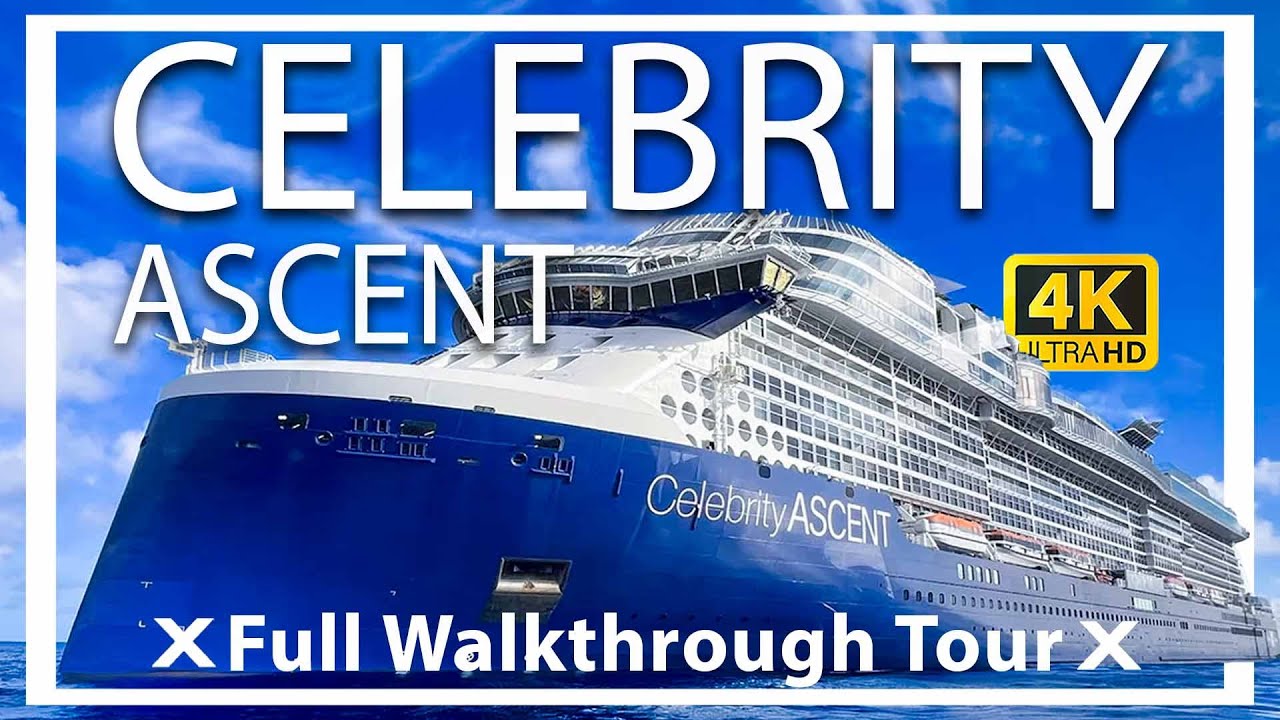The image features a blue and white cruise ship named Celebrity Ascent, prominently sailing on a blue ocean towards the lower left corner. The top part of the ship is white, lined with numerous windows, while the hull and bow are dark blue with the name "Celebrity Ascent" printed in white text on the side. The image appears to be a flyer or thumbnail for a YouTube video, indicating a detailed tour of the ship. Superimposed over the cruise ship is a small gold rectangle with the text "4K Ultra HD," and at the bottom of the image, in white text, it says "X, Full Walkthrough Tour X." The scene is set during the daytime, with a dark blue sky featuring white clouds.